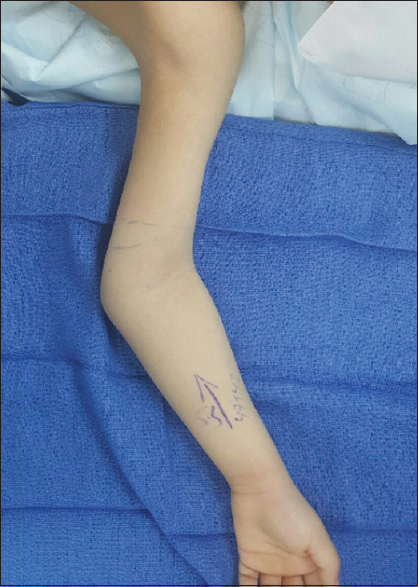The photograph captures the left arm of a child, poised in preparation for surgery. The thin, elongated limb is laid out atop blue gauze or a blanket, contrasting against the white linens and crumpled pillow of the gurney bed supporting the young patient. This bare arm features visible markings: a prominent purple arrow stretching from the wrist towards the elbow, indicating the intended site of incision, along with some accompanying letters and numbers that appear slightly smudged. The shoulder and armpit areas are just visible at the top of the image, while the hand is partially cut off at the bottom, showing only the palm and the first joints of the fingers. The overall relaxed positioning of the arm amid the surgical preps underscores the imminent medical procedure.